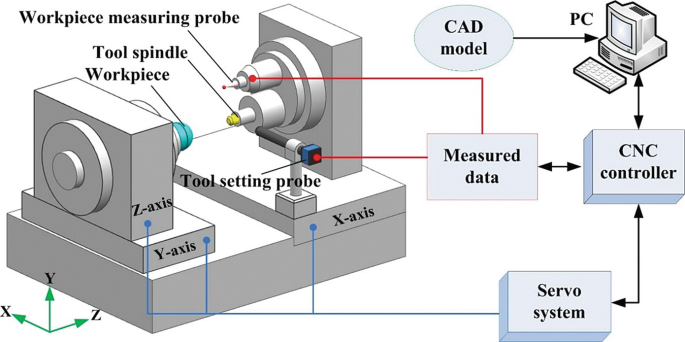The illustrated image showcases a detailed diagram of a measurement and control system, likely for a CNC machine setup. On the far left, there's a depiction of a device with several labeled components: a "Workpiece Measuring Probe" is identified near the top, alongside a "Tool Spindle Workpiece" shaded in aqua or teal. Further labels mark the "Tool Setting Probe," and the X, Y, and Z axes are clearly highlighted with corresponding arrows at the bottom left, illustrating their dimensional directions—X for width, Z for depth, and Y for height.

At the top center of the image, a bluish-gray circle labeled "CAD model" points down to a "PC." From the PC, arrows extend to a "CNC Controller," which has connections branching to "Measured Data" on the left and a "Servo System" below. The Servo System further links back to the X, Y, and Z axes, completing the control loop. The image illustrates how the CAD model is processed through the computer and the CNC controller, which then communicates with the Servo System to manage the various probes and axes for precise measurement and operation of the machine parts.